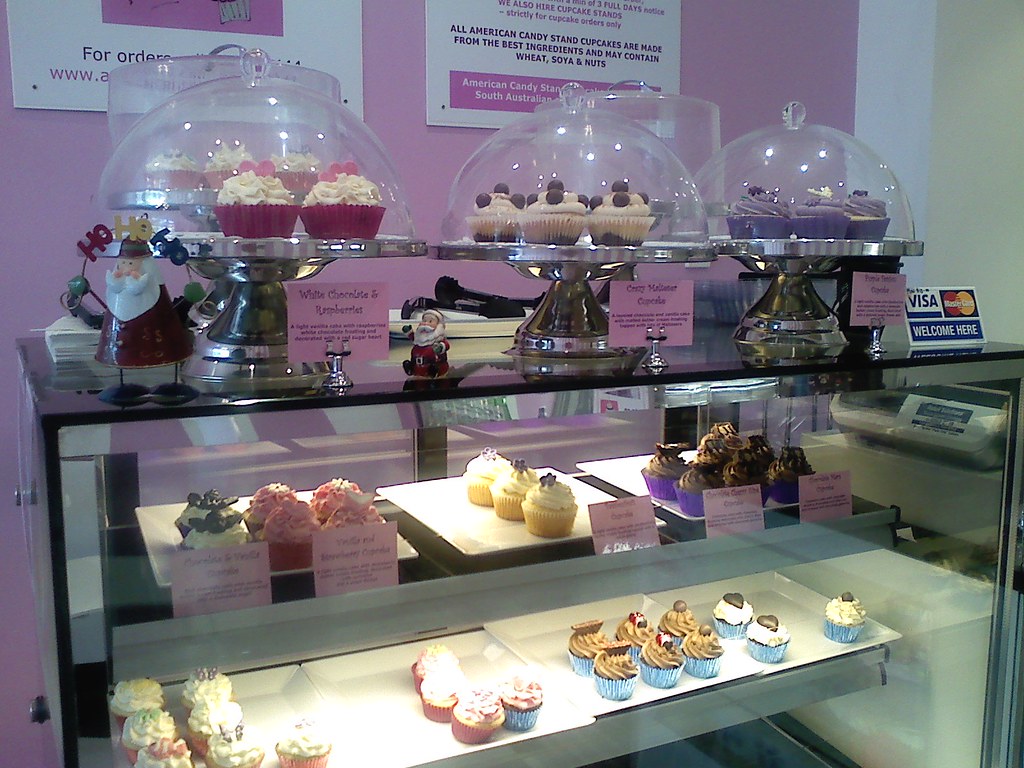In this image of a dessert shop, we see a glass display cabinet containing an array of cupcakes on two visible shelves. On the bottom shelf, there are four white trays, each holding different types of cupcakes. The two left trays feature pink cupcakes with white icing, while the right trays showcase blue cupcakes, one set with brown icing and toppings, and the other with white icing and chocolate toppings. The middle shelf contains three trays with cupcakes labeled by pink cards, though the labels are unreadable. The first tray has two cupcakes with white icing and chocolate toppings, alongside four pink-wrapped cupcakes with pink icing. The second tray holds three cupcakes with white topping and cream, while the third tray contains six cupcakes with purple wrappers, brownie-colored cream, and chocolate toppings.

Atop the cabinet, there are additional banquet dishes with glass domes, containing more cupcakes. Among the decorations, there are two Santa Claus figures, one on the right with the phrase "Ho Ho Ho" and another sitting in the center. The right side of the cabinet displays a Visa and MasterCard sign, and in the background, a pink wall adorned with white signs and posters. One poster mentions, "All American kindest and cupcakes are made from the best ingredients and may contain wheat, soy, and nuts." The display case itself is silver with white and black shelves, and scattered cupcakes in blue, red, yellow, and brown colors signify a busy day at the shop, with several trays already partially empty. The shop's register area is faintly visible through the glass on the right side of the cabinet.